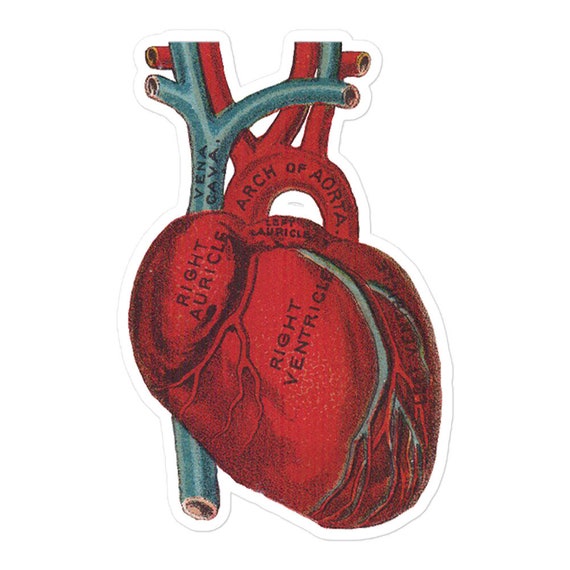This is an anatomically accurate illustration of the human heart, showcasing its various sections with labeled annotations directly on the respective parts. The heart is depicted in red and blue hues, with red labeling the right auricle, right ventricle, left auricle, left ventricle, and the arch of aorta, which is displayed as an arch above the heart. The blue sections highlight the vena cava and several veins. The image seems to have a sticker-like outline, giving it a slightly elevated, 3D appearance. The labels are in capital letters and the drawing has a rectangular portrait orientation, emphasizing the detailed anatomical features and the distinction between veins and arteries.